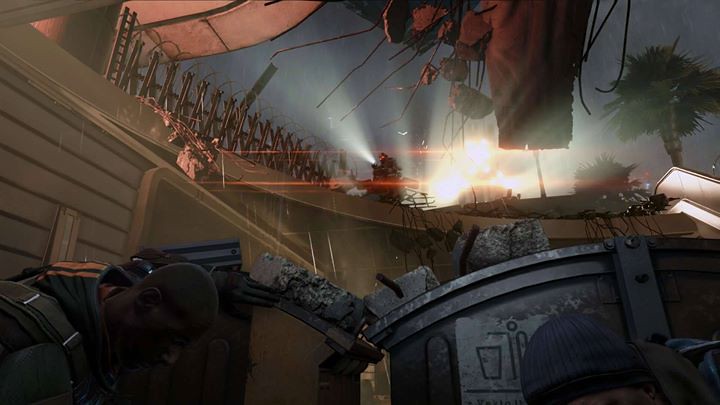The image depicts a dramatic scene, likely an illustration or painting, featuring a detailed setting and notable characters. Dominating the lower left corner is a bald black man, wearing a black coat with orange stripes and black gloves, with straps over his shoulders suggesting he's carrying a pack or gear. His hand is pressed against a wooden wall, which is part of a structure that resembles a boat's hull or the lower deck of a building with a hollow bottom and metal-framed doors. 

Above him, partly obscured by shadows, is another man, possibly a firefighter, identifiable by his attire and a bright white flashlight he holds, which illuminates the scene by shining the light up and to the left. This man wears a gray skullcap with a black elastic band. 

The setting is surrounded by brown wooden walls, possibly made of planks, indicative of a boat or a damaged building, as part of it appears open to the dark sky above. The top section of the image reveals the silhouettes of a few trees against the night sky, with various objects hanging or strewn about, adding to the chaotic atmosphere. The use of light and shadow, combined with the detailed textures, elevates the tension and precariousness of the scene, suggesting it depicts a moment of crisis or aftermath of destruction.